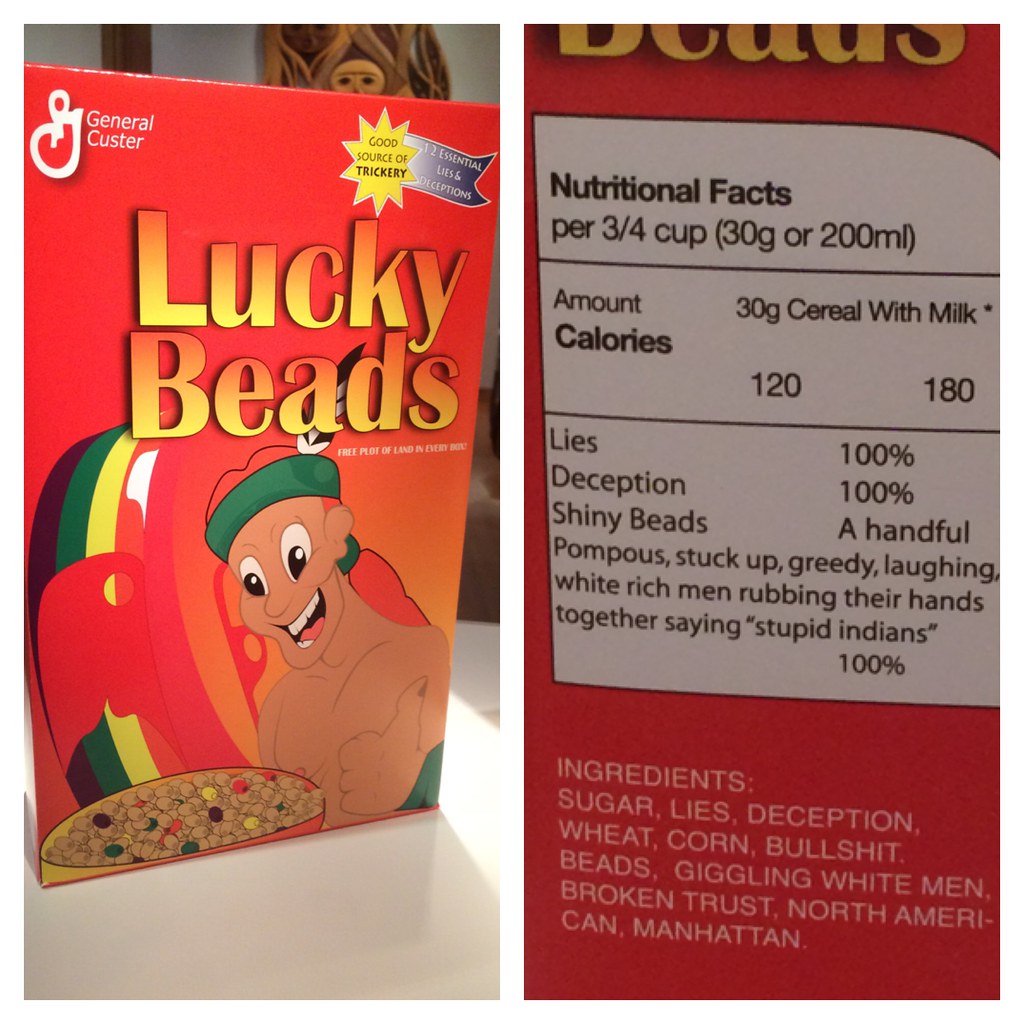This image is a parody product photo featuring two separate images side by side. The left image showcases the front of a cereal box labeled "Lucky Beads," clearly designed as a comedic spoof of the well-known "Lucky Charms" cereal. At the top left corner of the box, the name "General Custer" is displayed, while the top right corner humorously proclaims the product as a "Good Source of Trickery" with "12 Essential Lies and Deceptions." Dominating the front of the box, bold text spells out "Lucky Beads." Below this, a cheerful man with red hair and a single feather tucked into a bandana is pictured, giving a thumbs up with a wide, enthusiastic smile as he gazes at a bowl of cereal. 

The right image replicates the style of a typical Nutrition Facts label but with satirical content. The label lists calories along with exaggerated ingredients such as "Lies, 100%," "Deception, 100%," and "Shiny Beads, a Handful," maintaining the playful and mocking tone of the cereal box illustration. The overall design is clearly intended to be a humorous critique of sugary cereals and their marketing strategies.